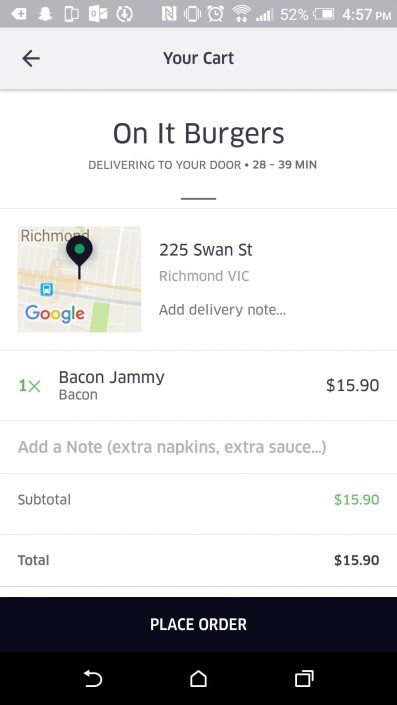The screenshot displays a smartphone screen showing the cart details from a food delivery app. At the top, the screen bears the heading "Your Cart" followed by “Onnit Burgers delivering to your door, 28 to 39 minutes” beneath it. The next section features a Google Maps pinpoint illustration indicating the restaurant's location, with the address listed as “225 Swan Street, Richmond, VIC” to its right. Below this, there is an option to “Add delivery note…” followed by the order summary. It shows an item: “Bacon Jammie” (one unit) priced at $15.90. The subtotal and total charges both amount to $15.90. At the very bottom, a black button with white text labeled “Place Order” is prominently displayed. The background of the screen is predominantly white. At the very bottom of the screen are three navigation icons: a back arrow, a home icon, and two overlapping squares.